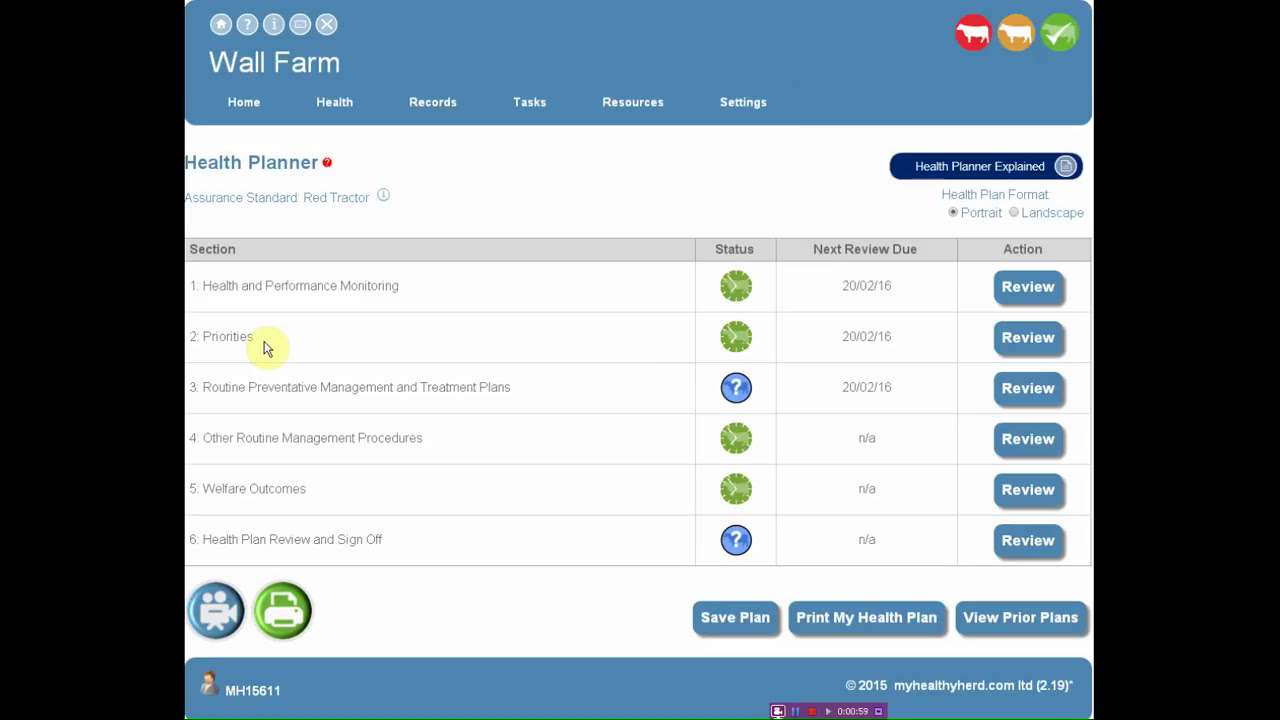The image is a detailed screenshot from a web or desktop application called "Wolf Arm." At the top of the interface, there are icons for Home, Help, Information, Chat, and Exit. Below these icons, the title "Wolf Arm" is displayed, followed by a navigation tab featuring six headers: Home, Health, Records, Tasks, Resources, and Settings. The user appears to be on the "Health Planner" section, indicated by a red dot beside that tab. The screen prominently displays the label "Assurance Standard Red Tracker" alongside a detailed information box titled "Health Planner Information Explained."

The central part of the screen contains a table with columns labeled Section, Status, Next Review Due, and Action. The table lists six sections: Health and Performance Monitoring, Priorities, Routine Prevention Management and Treatment Plans, Other Routine Management Procedures, Welfare Outcomes, and Health Plan Review and Sign Off. Each section is marked with a status symbol—a green clock face or a blue question mark—and includes review dates. The action for all sections is set to "Review."

In the upper right corner of the interface, there are icons of cows in different colors: red, green, and orange, with the green one marked by a check. The lower left corner features symbols of a blue camera and a green printer. The bottom of the screen includes buttons for Save Plan, Print My Health Plan, and View Prior Plans. The entire page is text-centric with a colorful, predominantly blue background, integrating the described icons and statuses seamlessly into the health management tool.